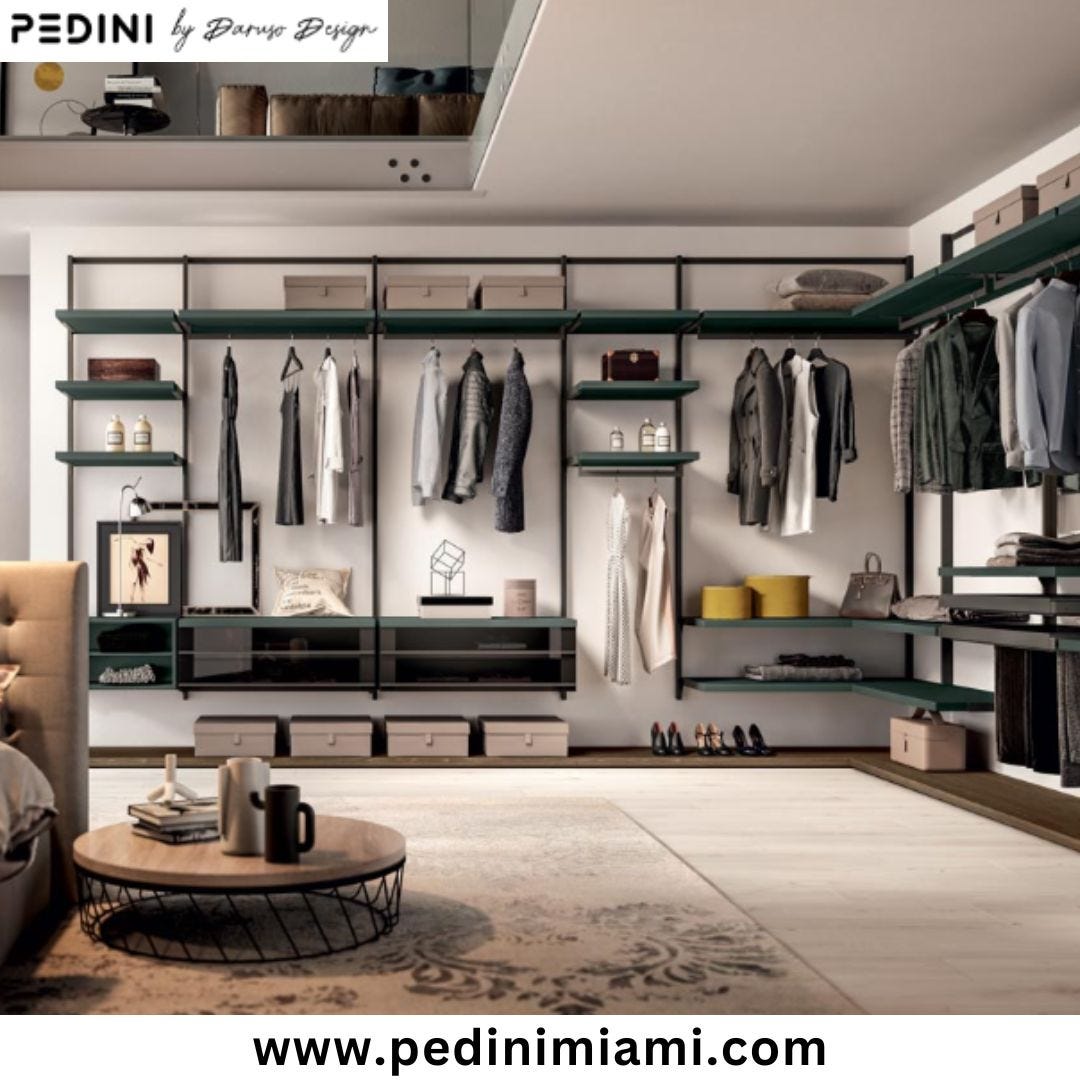This image features a large, organized wardrobe against a primarily white or slightly off-white wall, prominently displaying various clothing items. The wardrobe is composed of multiple sections and shelves, some of which are dark green in color. Each section contains a few carefully arranged clothing items, including dresses, jackets, blazers, coats, shirts, and pants. Toward the bottom of the wardrobe, there are several cream-colored shoeboxes and three pairs of high-heeled shoes. Additionally, there are hat boxes, a yellow hat box, purses, and storage boxes varying in shape, with some being square and others round.

The flooring beneath the wardrobe is a combination of cream-colored sections and a darker cream-colored patterned rug. On the left-hand side of the image, partially visible, is a tan chair with a tall back, facing forward, next to a wooden circular coffee table with a designed metal mesh base. Positioned on top of this table are a coffee cup and a coffee pot.

Text found within the image includes “Padini by Dario Design” in a stylized black font on a white background located at the top left corner. At the bottom center of the image, the website www.padinimiami.com is displayed in black text. The overall impression is that of a high-end, organized clothing store or a meticulously arranged wardrobe space.